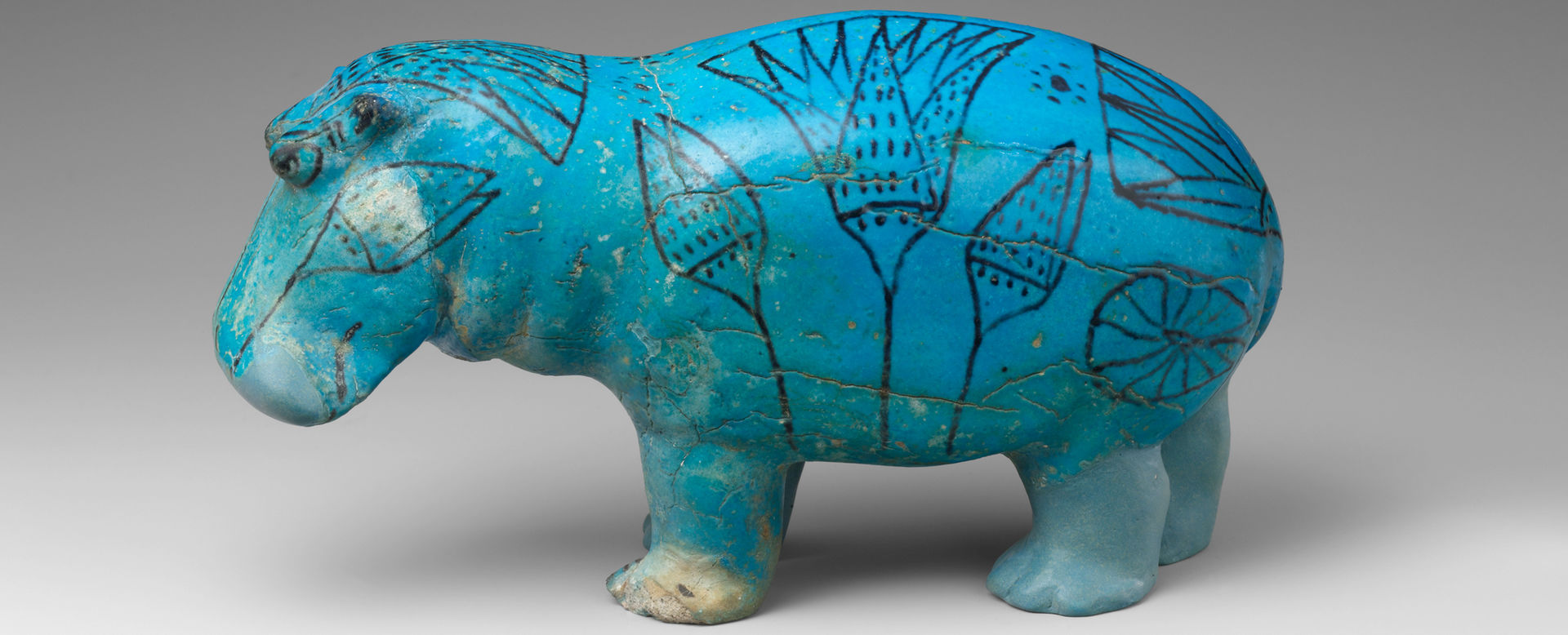This indoor image features a close-up of a blue, ceramic sculpture of a hippopotamus, possibly an antique or ancient piece of artwork. The sculpture stands on a white table against a white background, giving the image a clean and focused presentation. The artwork portrays a meticulously detailed hippopotamus, oriented with its head facing the left side of the image and its tail to the right. The figure exhibits a two-tone blue coloration: a lighter blue at the front, extending to the legs, and a darker blue at the back. Intricate black designs, reminiscent of Aztec or indigenous patterns, adorn the face, sides, and rear of the hippopotamus, adding a layer of cultural significance. Notably, the sculpture shows signs of wear, with cracks visible from the back to the front, suggesting its age and possibly its historical value, which might indicate it is on display in a museum or gallery setting. The overall presentation, complete with subtle shadowing, emphasizes the artifact's intricate details and historical aura.